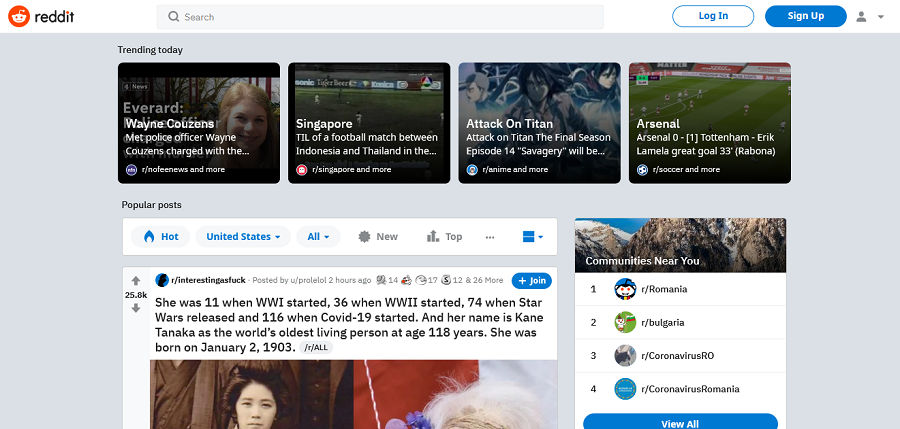This is a detailed screenshot of the Reddit website interface. At the top, there is a white navigation bar. On the upper left corner, the recognizable Reddit logo is prominently displayed, featuring a red circle with a white alien head icon. To the right of the logo is a light gray search field decorated with a small, darker gray magnifying glass icon on the left side, and the placeholder text "search" in gray font to the right.

Continuing rightward, there are two prominent buttons: one white with blue font labeled "log in" and another blue with white font labeled "sign up." Further to the right of these buttons, there is a small silhouette icon of a human figure.

Beneath this navigation bar, the content section begins with a gray background and the phrase “Trending Today” in bold black font at the top. Below this header, there are four side-by-side selections highlighting trending topics. The first trending item reads, "Wayne Cousins: Met Police officer Wayne Cousins charged with…". The second item states, "Singapore: TIL of a football match between Indonesia and Thailand in the…". The third trending topic is about "Attack on Titan: Attack on Titan the final season episode 14. Savagery will be…". 

(Please note: The "dot-dot-dot" suggests that the text is truncated and not fully visible in the screenshot).